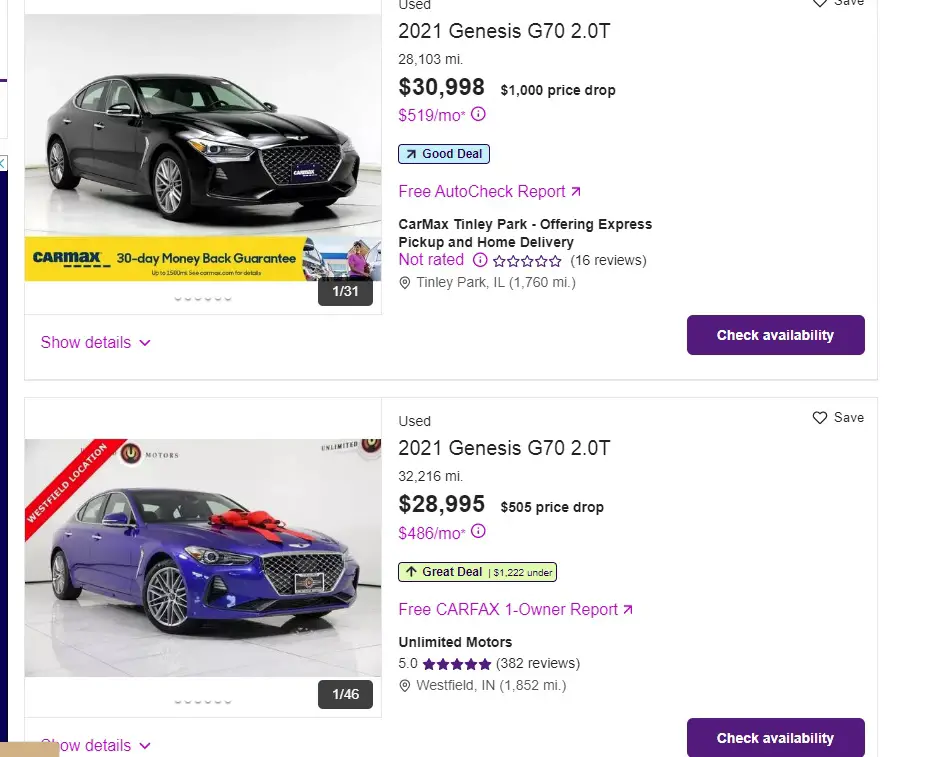This square-shaped photo depicts search results for vehicles from various websites, possibly including CarMax. The image showcases two search results formatted against a white background, each featuring landscape-oriented photos that are wider than they are tall.

The first search result displays a black 2021 Genesis G70 2.0 Turbo with over 28,000 miles, priced at $30,998. The monthly payment is highlighted in purple, and there is a link to a free AutoCheck report in pink next to it. Below the car details is a yellow CarMax banner with blue letters, indicating that this is picture 1 out of 31. A pink drop-down box reveals more details about the car, and a rectangular purple box labeled "Check Availability" with white font is positioned to the left.

The second search result features a blue 2021 Genesis G70 2.0 Turbo with 32,000 miles, available for $28,995. A green box with an upward-pointing arrow labeled "Great Deal" suggests the price is lower than usual. This listing is marked as image 1 out of 46 and boasts a 5.0 rating from the seller. Similar to the first listing, there is a purple "Check Availability" box.